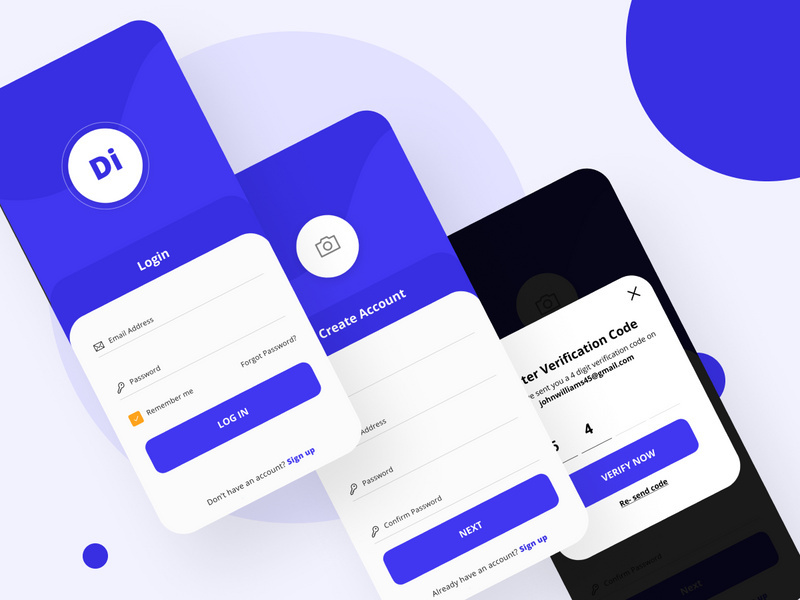The image features a pale purple background adorned with various geometric shapes, including a light lavender circle and a purplish-blue half-circle situated at the top right. There's a small purple circle positioned just below one of the main elements, and a blue-purple circle located at the bottom left. In the center of the image, laid out diagonally, are three rectangular objects resembling smartphone screens.

The top screen displays a login page with the following details:
- A white circle with the letters "Di"
- Form fields labeled "Email Address" and "Password"
- A "Remember Me" option with an orange square and a white checkmark inside it
- A "Forgot Password" link
- A purple "Log In" button with white text
- A prompt saying "Don't have an account? Sign Up" in purple text with a capital "S"

The middle screen shows a create account page with:
- An icon depicting a camera
- Fields for "Email Address," "Password," and "Confirm Password"
- A "Next" button
- A note saying "Already have an account? Sign Up"

The bottom screen, partially obscured by the middle one, displays:
- A black background with a prompt to "Enter Verification Code" along with four spaces for code digits
- A partially visible code where the second digit is '4'
- Options to "Verify Now" or "Resend Code"